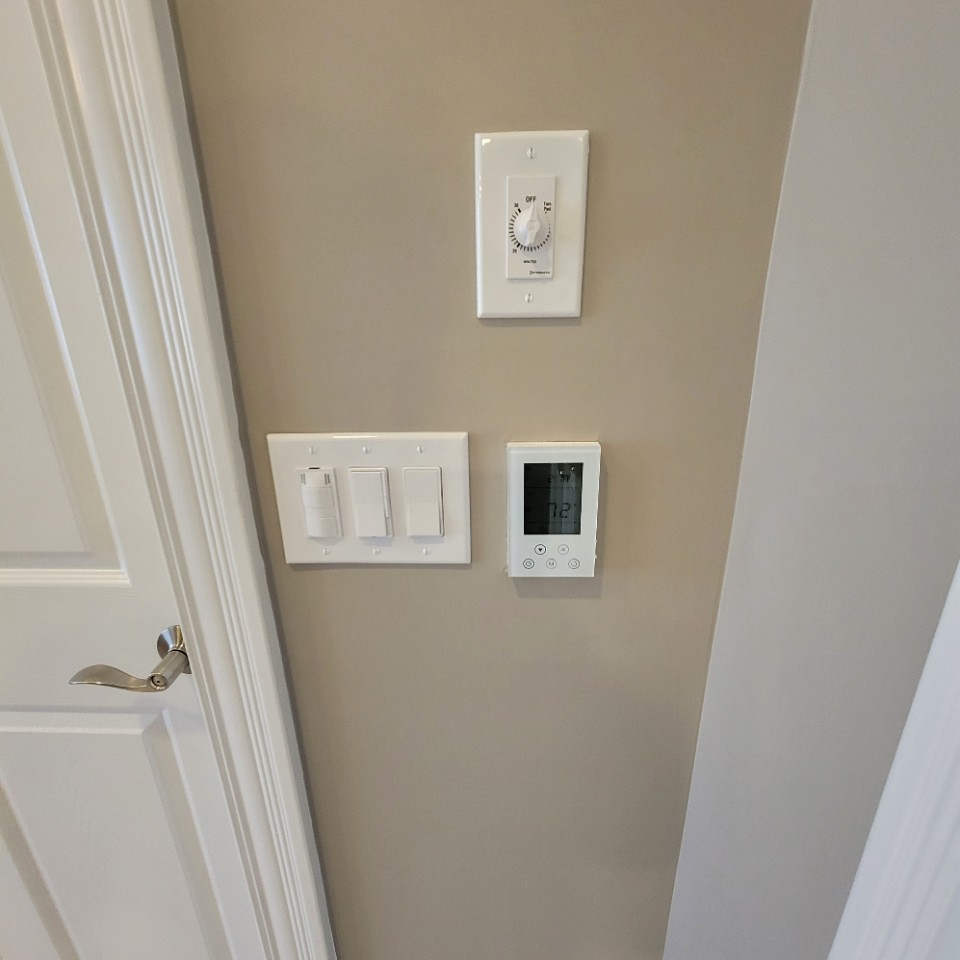In this image, the left side features a white door with a sleek silver lever-style door handle. Adjacent to the door, the beige wall hosts several fixtures. There is a dimmer switch with an integrated timer, a set of three flat push-button light switches, and a digital thermostat displaying temperature in a small, button-equipped box. Further to the right, a section of the wall above a likely shower curtain rod is visible, suggesting the setting is a bathroom. The various controls on the wall likely pertain to lighting and climate adjustments within the room, offering practical convenience near the shower area.